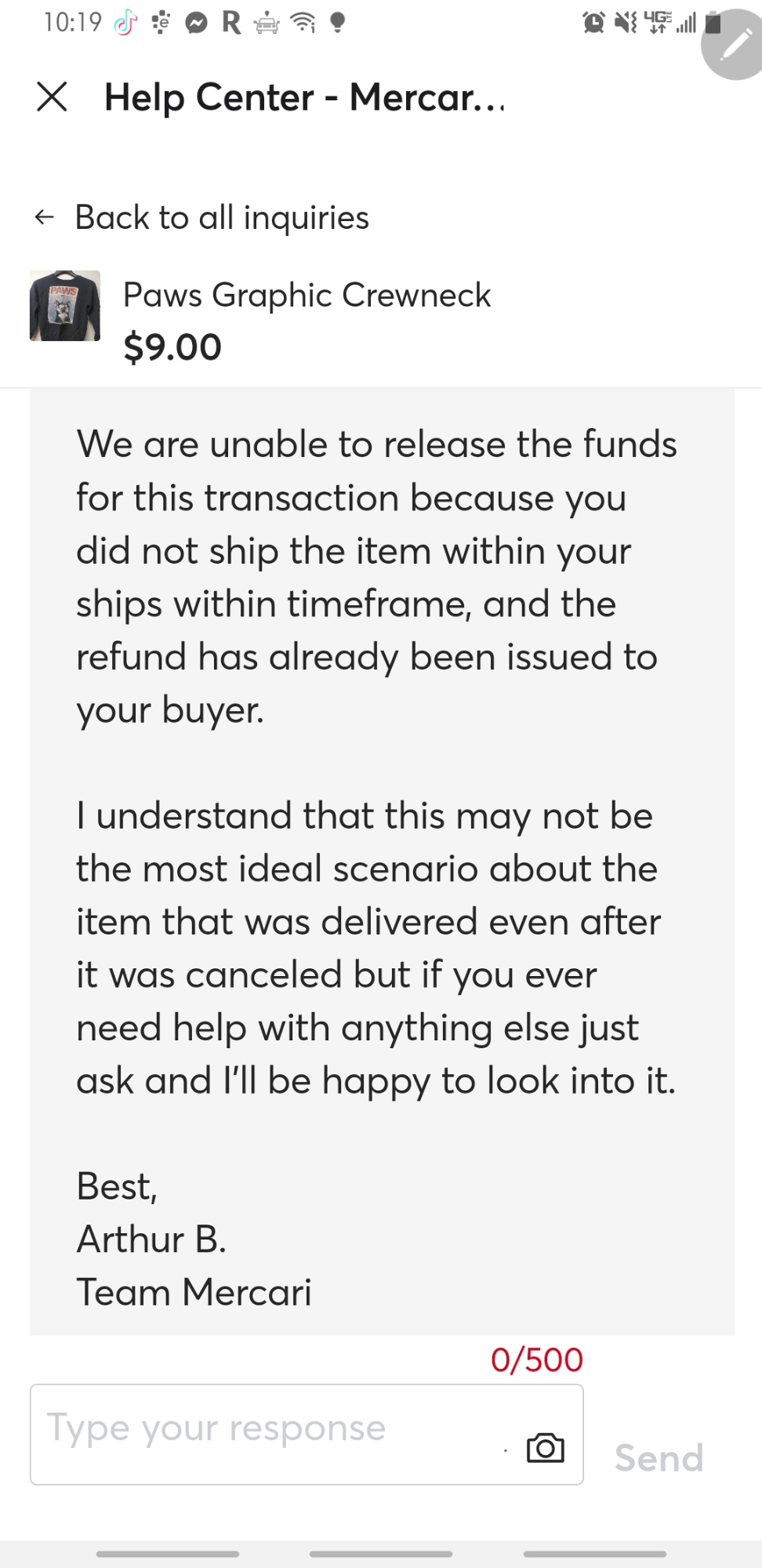This image is a screenshot captured from either a tablet or a smartphone. The status bar at the top displays various icons: the time "10:19," a TikTok logo, a crossed circle with dark boxes, the Facebook Messenger icon, an "R," a car, a WiFi signal with an exclamation mark (indicating no connection), a light bulb, a clock, a muted speaker, "4G," a cell phone signal strength indicator, and a battery icon. Additionally, there is a dark grey circle with a pen icon, indicating that the pen from the note has been removed.

Just below the status bar, there is an "X" icon followed by bold black text that reads "Help Center - MERCAR..." suggesting the text is cut off but likely refers to "Mercari." On the right side, a black arrow points left with the text "Back to all inquiries." The main content displays a black t-shirt featuring red text and a blue background, presumably depicting a black and white Husky dog. To the right, in bold black text, it reads "Paul's Graphic Crew Neck $9."

Below this, a message from the company Mercari is shown: "We are unable to release the funds for the transaction because you did not ship the item within your ship's within time frame and the refund has already been issued to your buyer. I understand that this may not be the most ideal scenario about the item that was delivered even after it was cancelled, but if you ever need help with anything else just ask and I'll be happy to look into it. Best, Arthur B. Team Mercari."

At the bottom of the screenshot, there is a "0 out of 500" character count in red, a text box labeled "Type your response" in light grey, a camera icon, and a grey "Send" button.